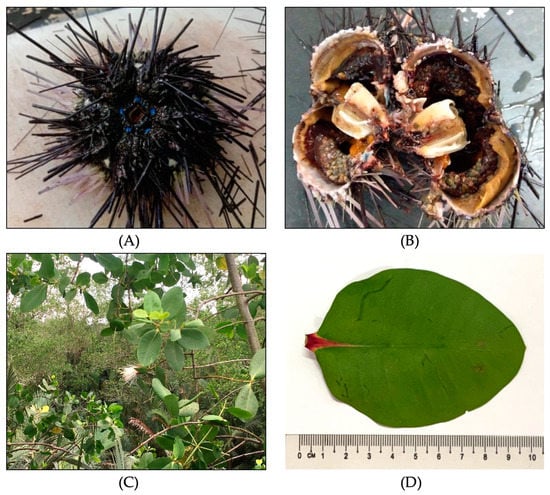The image is a square collage divided into four quadrants, each featuring a distinct subject and labeled with letters in parentheses. The top left quadrant (A) showcases a black sea urchin with broken spines and blue dots near its mouth, set against a white background. The top right quadrant (B) reveals a cross-section of a sea urchin, exposing its hollow cavity and central muscular structure, surrounded by loose spines, on a gray background. The bottom left quadrant (C) presents a lush, forest-like scene possibly depicting mangroves, with close-up views of branches, leaves, and tall grass. The bottom right quadrant (D) displays a single, green oval leaf with a red base, positioned sideways with the stem on the left, on a white background alongside a 10-centimeter ruler. Each quadrant is outlined in black, except for the bottom right.